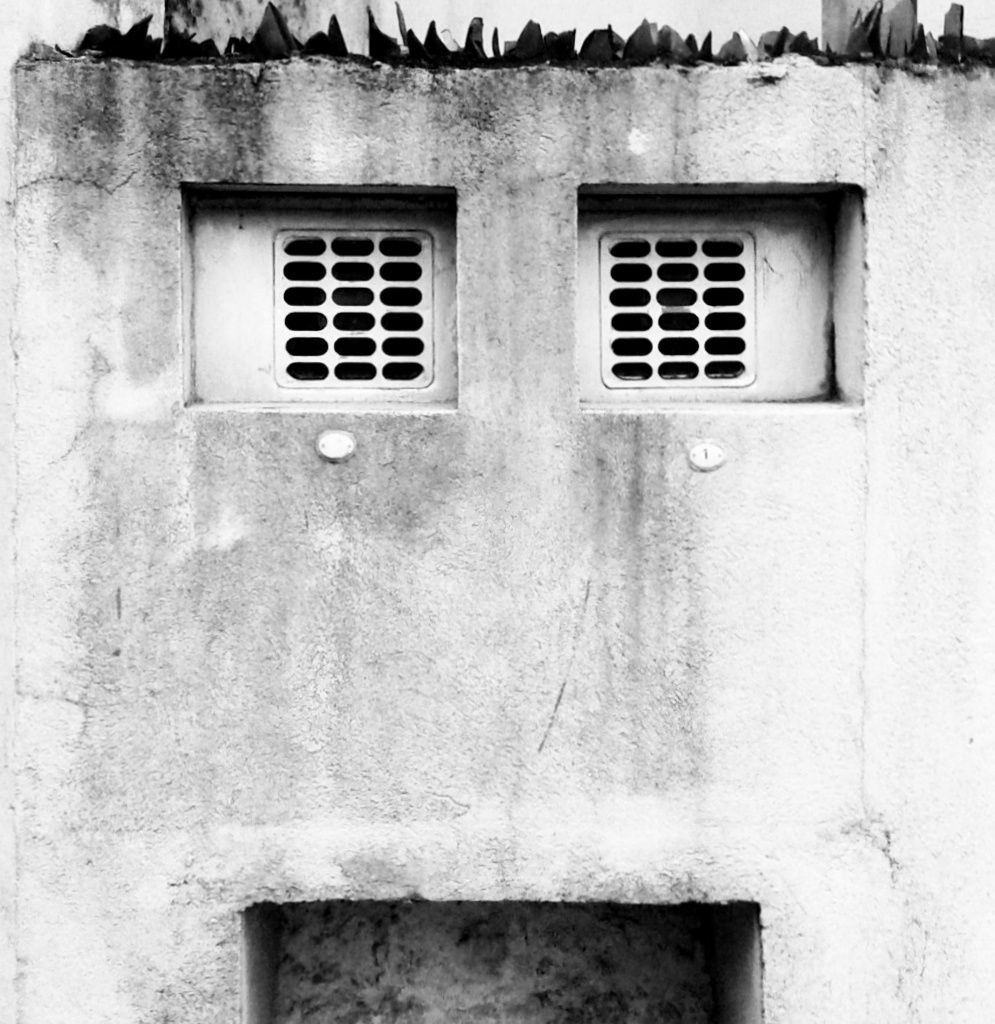This black and white photograph captures an old cement wall that intriguingly resembles a human face. The image prominently features two upper air vents or ducts, situated like eyes, with a grill-like pattern. Below these vents are two oblong shapes affixed to the building, appearing as if they could be cheeks. Atmospheric cracks and dirt cover the surface of the wall, adding texture and depth. Near the bottom of the photo, the top foot of a darkened doorway or indentation is visible, resembling a mouth. This artistic composition is enhanced by jagged, glass-like vegetation on the roof, adding a unique, almost protective layer to the top of the structure. The photograph, devoid of color, emphasizes the facial mimicry of the architectural elements, inviting viewers to see the wall as more than just brick and mortar, but as a silent observer in the form of a robot-like face.